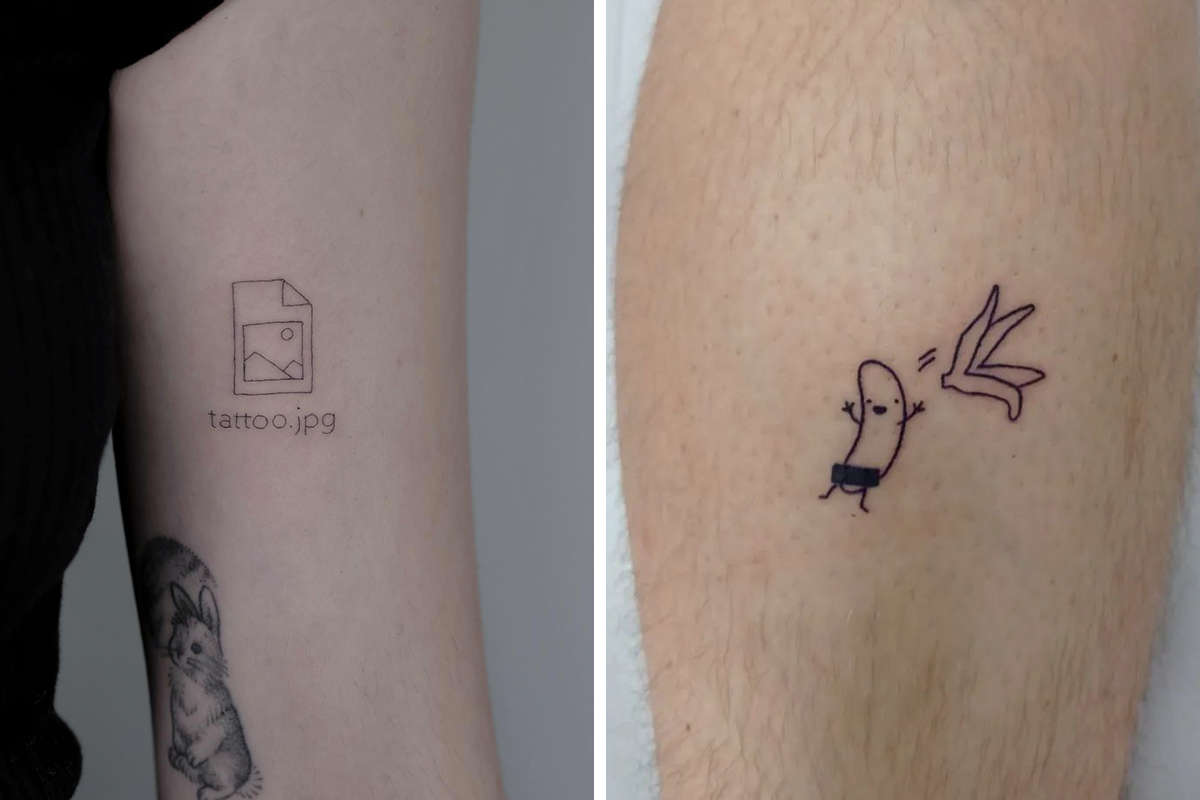The image is divided into two adjoining photographs, each showcasing a different tattoo on what appears to be white-skinned individuals. The left photograph features a person's upper arm, partially clad in a black t-shirt. Centrally located on the arm is a tattoo resembling a digital image file, complete with a folded corner and an icon depicting two hills and a sun, above the text "tattoo.jpg." Below and slightly to the left of this tattoo is another black-and-white tattoo of a rabbit. The right photograph focuses on a person's calf, which has been shaved around the tattoo area. This tattoo portrays an animated banana with arms, legs, and a smiley face, humorously flinging its peel, with a black censor bar covering parts of it. The background in the left image is gray, while the background in the right image is white.